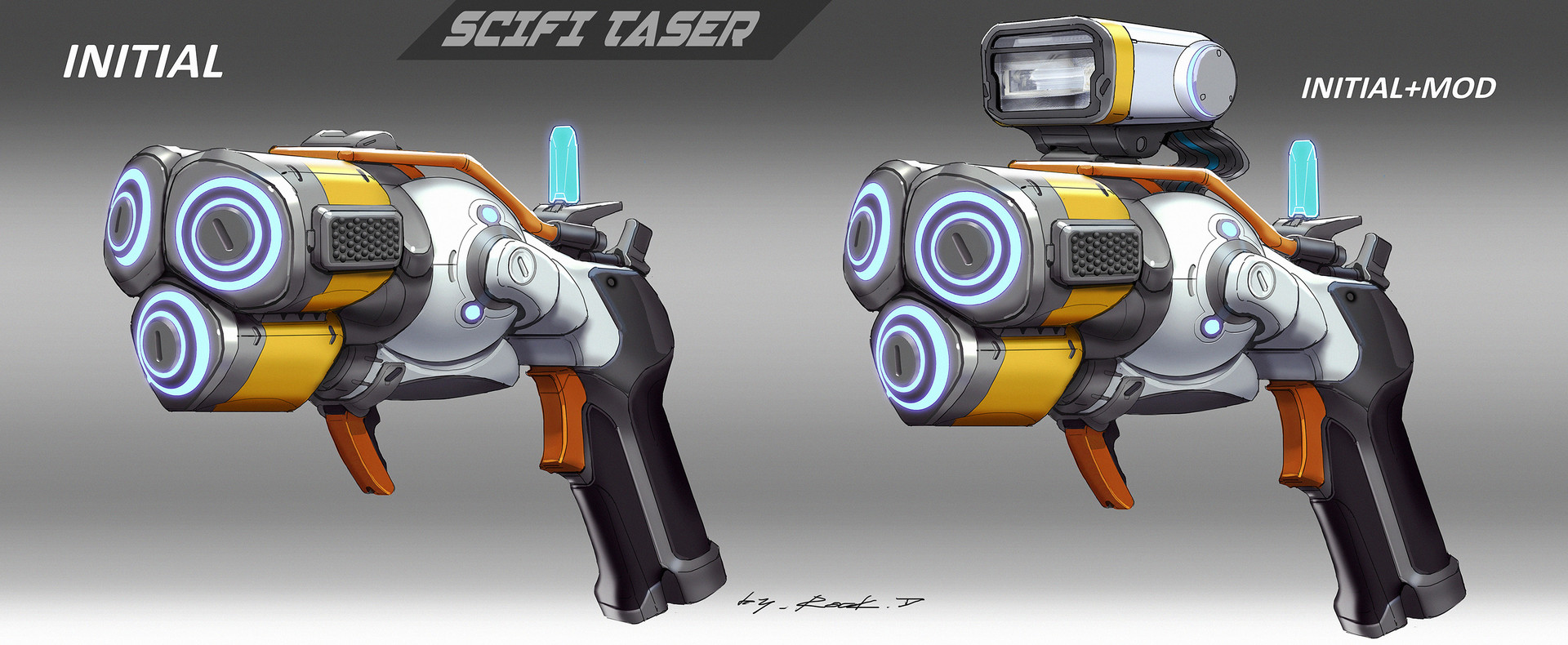The image depicts two identical-looking sci-fi taser guns set against a grey gradient background. Both tasers are presented upright with an overall cartoonish style, likely signifying prototype models. Each gun features a black handle with a pistol grip, a blue trigger, three yellow cylinders with blue tips likely indicating the taser mechanism, and two distinctive orange protrusions on either side. The key difference between the two is an additional piece of equipment on top of the taser on the right, which resembles an automatic flash or a projector. The taser on the left is labeled "initial," while the one on the right is marked "initial plus mod." Above the tasers, the text "Sci-Fi Taser" is displayed, and at the bottom, there's an unreadable cursive signature.